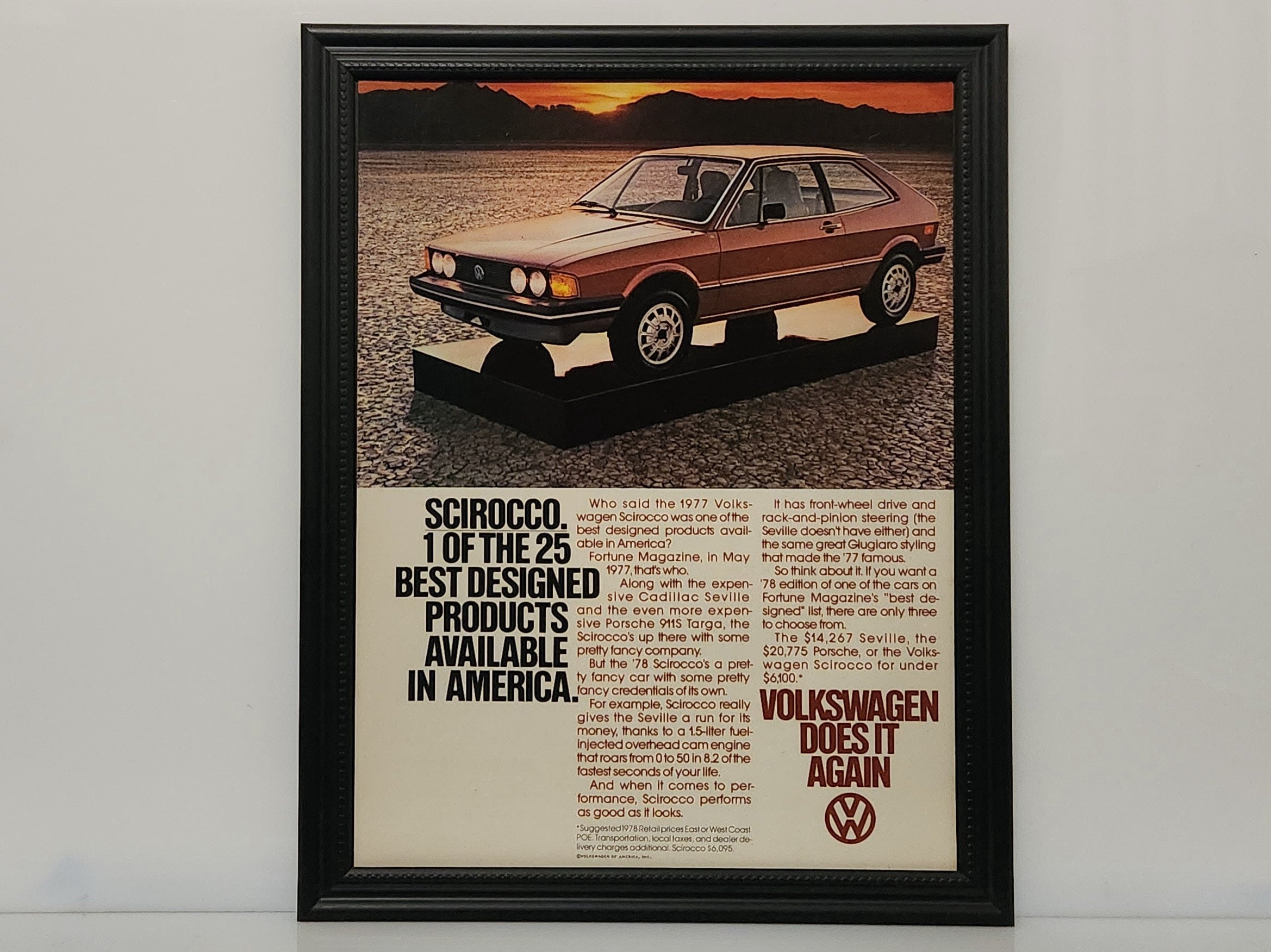The image depicts a meticulously framed vintage advertisement for a Volkswagen Scirocco, circa the late 1970s. The frame is black and thick, with a carved wooden texture, positioned against a light gray wall and resting on a white floor. The advertisement itself is divided into two distinct sections. 

The top half showcases a red Volkswagen Scirocco, a two-door hatchback, perched on a black pedestal that appears to be set in a coastal desert landscape. The scene features a dark brown stone ground that transitions into the distant silhouette of mountains against an orange sunset sky.

The bottom half of the image is a light cream color, featuring three columns of text. The left column, in bold black capital letters, reads: "SCIROCCO, one of the 25 best designed products available in America." The center and right columns consist of smaller, reddish-brown text in paragraph form, which is too small to read in detail. Adjacent to this text, towards the bottom right side of the image, the bold statement "Volkswagen does it again" is featured, accompanied by the Volkswagen logo.

Overall, this detailed photograph captures not only the elegance of the vintage car but also the nostalgic charm of the era, framed and presented as a prized piece of automotive history.